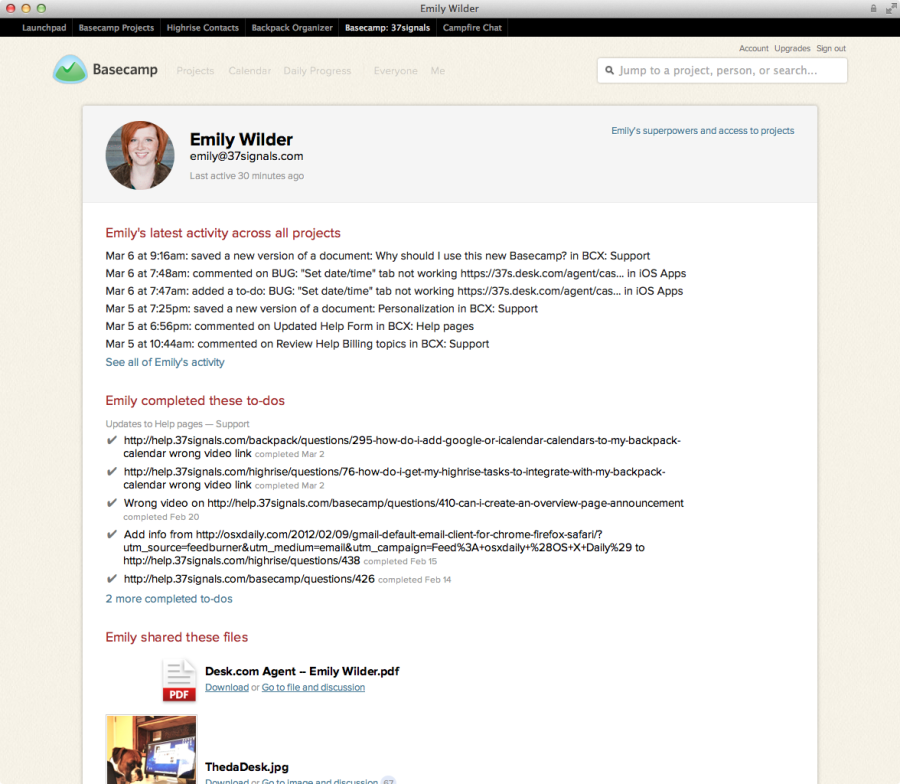The image displays a Mac screen with the typical red, yellow, and green buttons for close, minimize, and maximize in the upper left corner. The menu bar prominently displays the name "Emily Wilder" at the center. Below the menu bar are several menu options.

The main content of the screen appears to be a Basecamp interface, likely a webpage or document. On the far right, there is a search field labeled "Jump to a project, person, or search."

The upper left part of the content area features a photograph of Emily Wilder, with her name and email address displayed to the right of her photo. Below this, in red font, it says, "Emily's latest activity across all projects," followed by a list of dates and activities.

Further down, another red heading reads, "Emily completed these to-dos," listing several tasks, each marked with a check indicating completion.

At the bottom of the page, the section titled "Emily shared these files" appears, showing various files she has shared. The project names, to-dos, and file names are displayed in black font, emphasizing the contrast with the red headings.